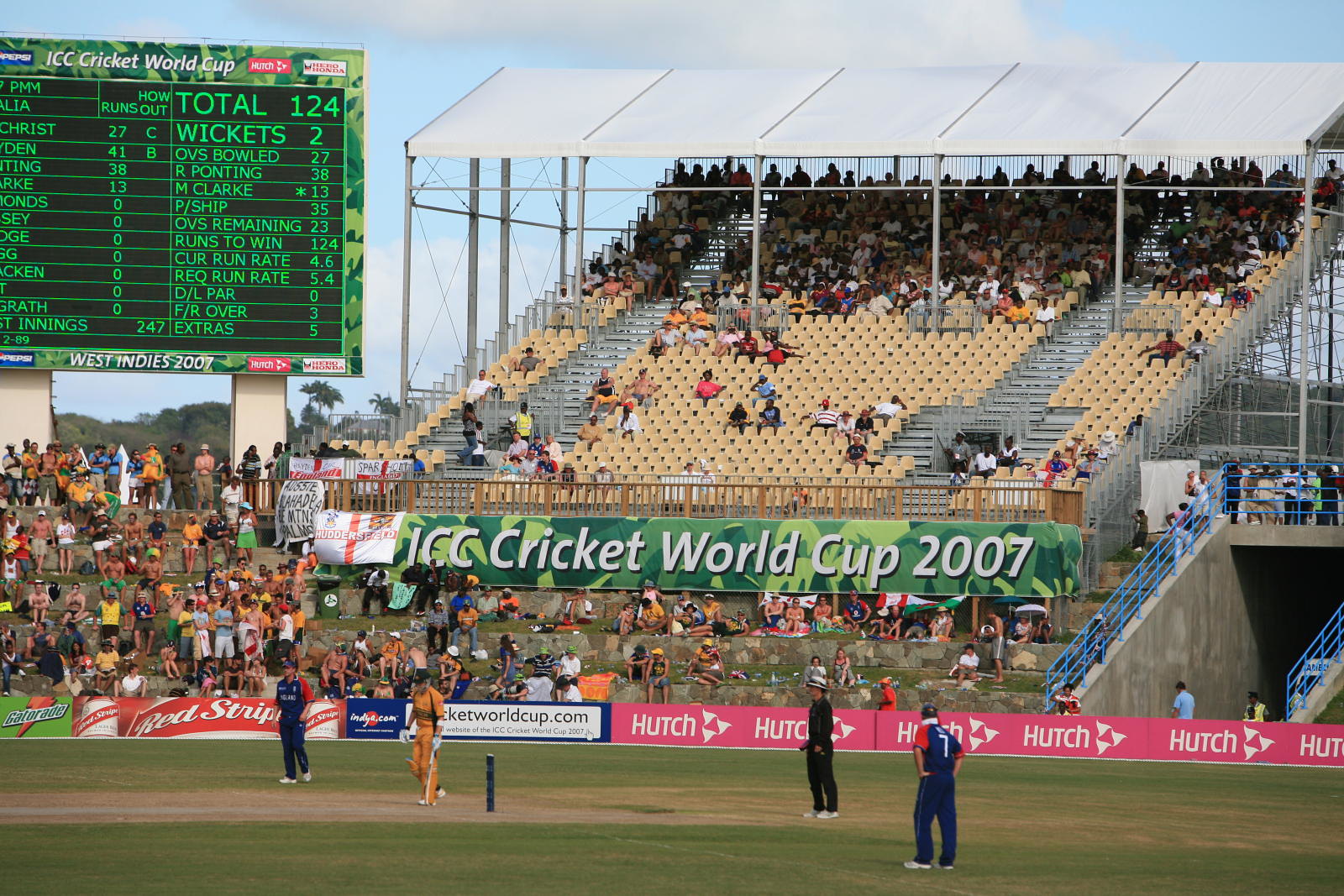This image captures the atmosphere of a cricket game at the ICC Cricket World Cup 2007. Dominating the scene is a large, green banner that reads "ICC Cricket World Cup 2007." The photograph is filled with the excitement of a live match in a vast stadium. The lush grass field is the focal point, with a few cricket players in action: two in blue uniforms with red sleeves, one in a yellowish gold uniform, and a referee dressed in black. Surrounding the field are various advertising banners for sponsors such as Hutch, Gatorade, Red Stripe, and TicketWorldCup.com. The scoreboard in the upper left corner displays a total of 124 wickets, along with player names and various statistics, framed by green text.

The stadium itself features stone bleachers divided into three sections, mostly occupied by spectators concentrated in the center. Above the seating area, a roof covered by a white tarp provides shade. In addition to the seating behind the players, a cement entranceway with a blue fence is visible to the right. The backdrop of the scene is a bright blue sky dotted with white clouds, encapsulating the lively and vibrant atmosphere of the tournament. Overall, this image offers a dynamic and detailed glimpse into the excitement of the ICC Cricket World Cup 2007.